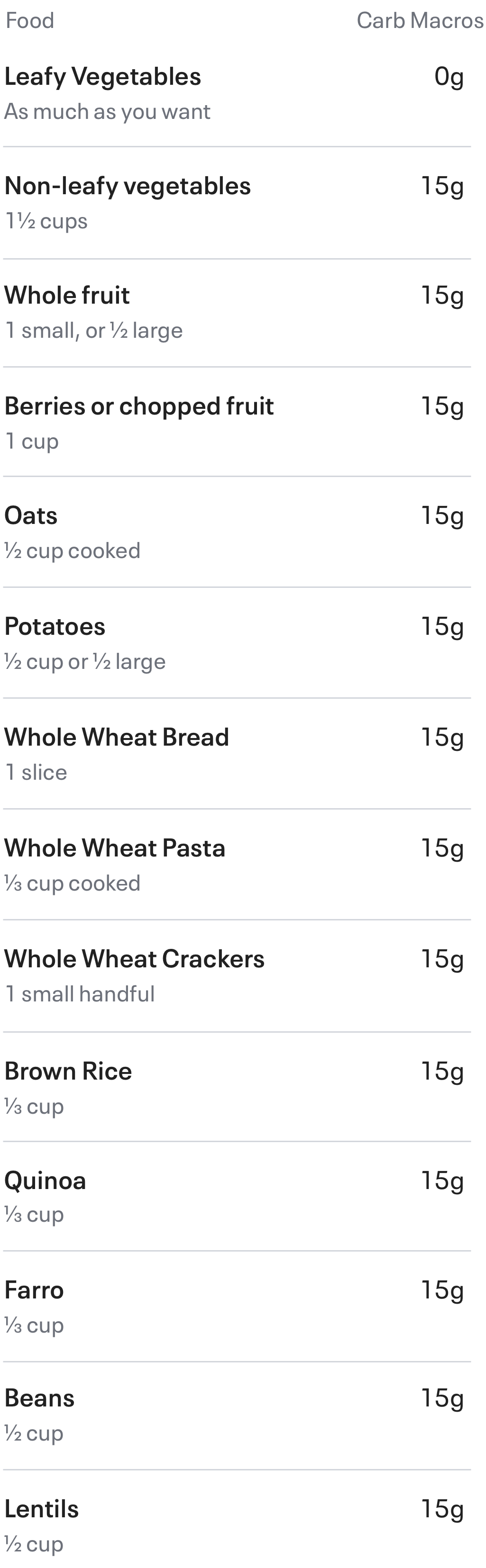The screenshot, set against a white background, comprehensively lists various foods and their corresponding carbohydrate macros. The breakdown is as follows:

- **Leafy Vegetables**: As much as desired, 0 grams of carbs.
- **Non-Leafy Vegetables**: 1.5 cups, 15 grams of carbs.
- **Whole Fruit**: 1 small or 1/2 large, 15 grams of carbs.
- **Berries or Chopped Fruit**: 1 cup, 15 grams of carbs.
- **Oats**: 1/2 cup cooked, 15 grams of carbs.
- **Potatoes**: 1/2 cup or 1/2 large, 15 grams of carbs.
- **Whole Wheat Bread**: 1 slice, 15 grams of carbs.
- **Whole Wheat Pasta**: 1/3 cup cooked, 15 grams of carbs.
- **Whole Wheat Crackers**: 1 small handful, 15 grams of carbs.
- **Brown Rice**: 1/2 cup, 15 grams of carbs.
- **Quinoa**: 1/2 cup, or 1/3 cup cooked, 15 grams of carbs.
- **Farro**: 1/2 cup, 15 grams of carbs.
- **Beans**: 1/2 cup, 15 grams of carbs.
- **Lentils**: 1/2 cup, 15 grams of carbs.

This detailed breakdown presents an easy-to-understand guide for managing carbohydrate intake through various food options.